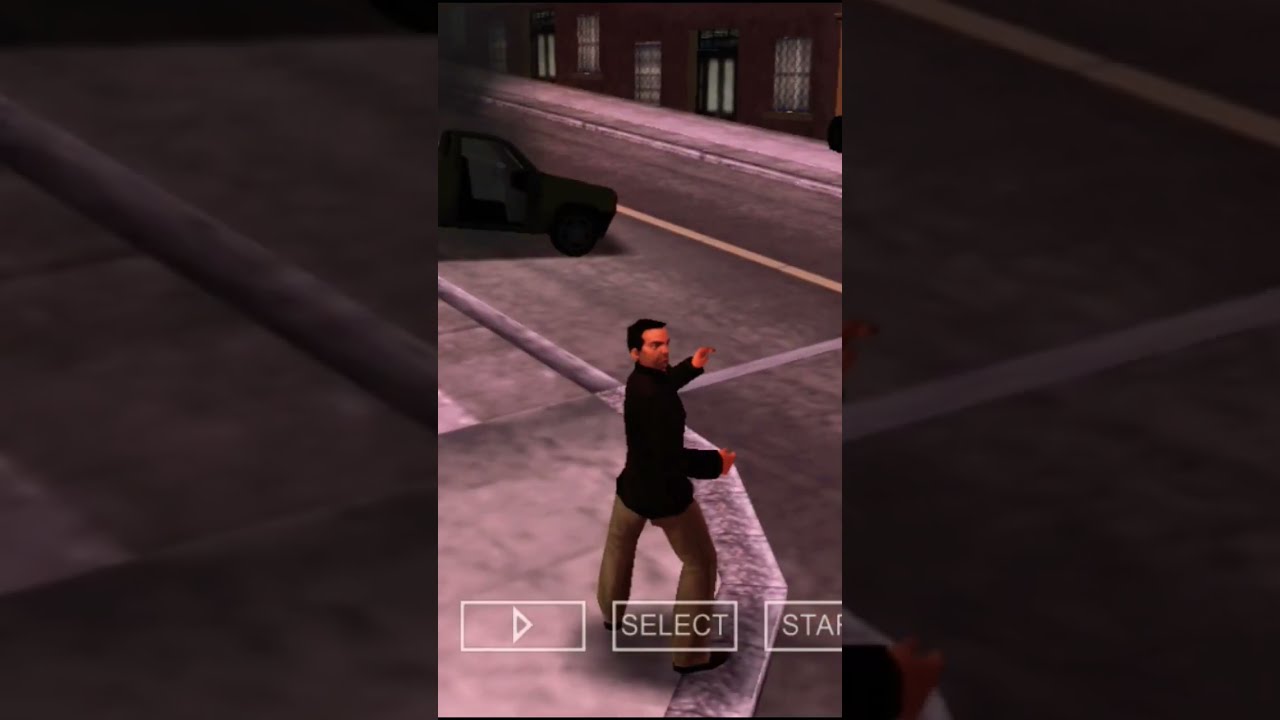The image appears to be a screenshot from an older Grand Theft Auto video game, likely from the early 2000s, characterized by its blocky, low-poly graphics. The central figure is a Caucasian male with short dark hair, wearing a black shirt and brown pants. He stands at the corner of a sidewalk, one foot on the curb and the other on the pavement, positioned with his legs slightly apart. His body is oriented facing away from the camera, but his head is turned to his right, and his arms are raised as if making a threatening gesture or on guard. About 25 feet away from him, there is a burnt-out vehicle, black and charred, with smoke emanating from the top and its doors fully open, parked crookedly on the street. The road curves around a corner and is slightly elevated, allowing a view of the top of a nearby building with brown, windowed facades. At the bottom of the image, partial game interface elements are visible, including a play button, a select button, and a blurred "start" button, indicating the screen's functional overlay.